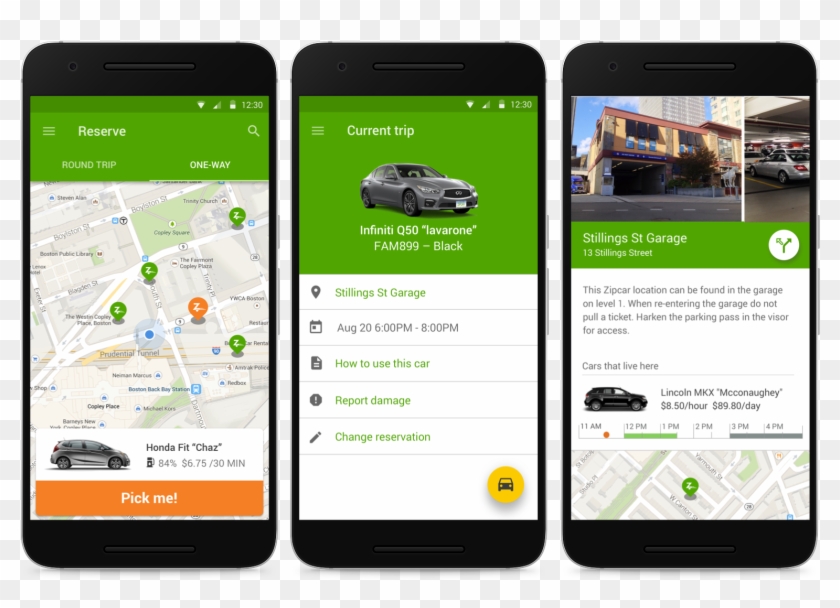The image captures a detailed interface of a car-sharing mobile application displayed on several cell phones.

The first screen of the app shows essential phone indicators, like time, battery life, and connection status. The app interface highlights a section for reserving cars, offering "Round Trip" and "One Way" options. Green locations indicate available retail locations, while one specific orange marker relates to a car listed as "Honda Fit Chaz." This car's image is displayed, accompanied by a "Pick Me" option and an orange bar with an exclamation point reading "Current Trip." Additional details include an Infiniti Q50 available at Stillings St. Garage from August 20th, 6 to 8 PM, with options to "How to use this car," "Report damage," and "Change reservation."

Another screen reveals an image of the Stillings St. Garage, highlighting its street address and the surrounding tan-colored skyscrapers. The garage's interior view displays a silver Lincoln MKX with rental rates specified as $8.50 per hour and $89.80 per day. A navigational map is also visible at the bottom of this screen. The application showcases a yellow circle icon with a car in the center, emphasizing the app's car-sharing service theme.